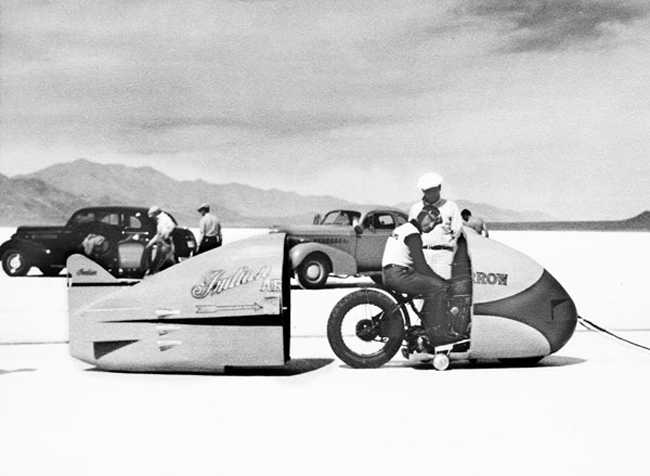This black-and-white photograph, possibly from the 1940s, depicts a scene on what appears to be the Bonneville Salt Flats. In the foreground, a man is seated on a motorcycle that is positioned in the middle of a two-part vehicle resembling a rocket. The front part of the motorcycle is encased in a rounded, rocket-shaped cone, and the rear section lies to the left, also designed to complete the rocket appearance. The motorcycle's single exposed wheel is visible, and the man seated has goggles on his forehead, wearing a white short-sleeved t-shirt over a black long-sleeved shirt with dark jeans.

Nearby, another man, dressed entirely in white—long-sleeved shirt, pants, and hat—is standing behind the seated man, possibly acting as a mechanic. Inscribed on the hull of the vehicle are the words "Julian" and "RROWR." 

In the background, two cars from the 1940s can be seen: one is a black sedan, and the other is a gray sedan. Two men stand in front of the black sedan, examining a similar type of vehicle. The scene is set against the backdrop of a mountain range with a gray, cloudy sky above, and the ground underfoot is the characteristic white surface of the salt flats, enhancing the stark contrast of the entire setting.